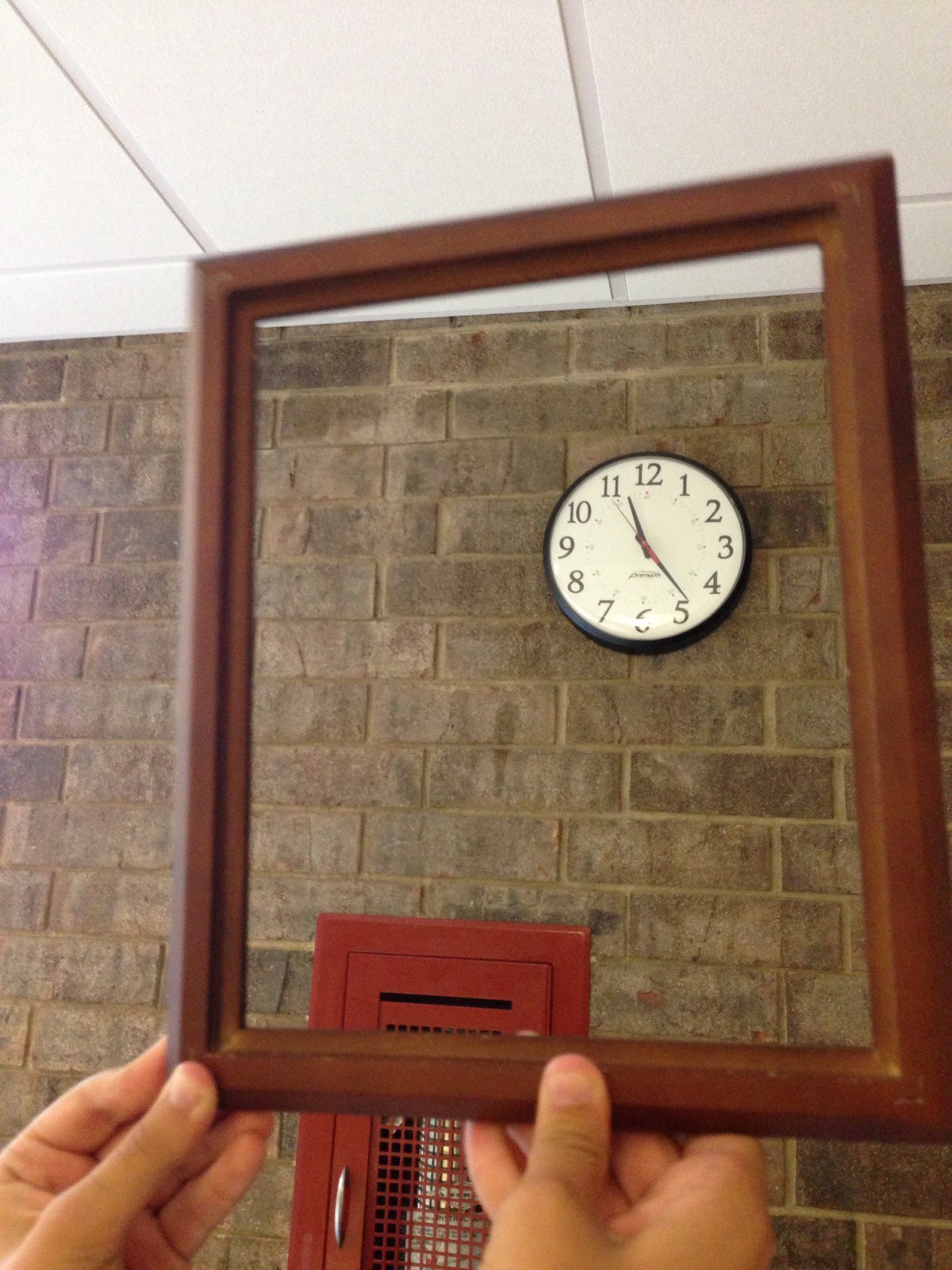This image, captured in portrait mode, features an intricately detailed scene centering on a white-faced clock with red hands and a black trim, positioned on an unpainted brown brick wall. Two thick-fingered, Caucasian male hands hold an empty reddish-brown wooden frame close to the camera, creatively giving the illusion that the clock is framed. The white, polystyrene drop ceiling creates a clean contrast above the brick wall. Below the clock and frame, a piece of furniture is partially hidden, identifiable by its red mesh front and a long silver handle, suggesting it might house a fire extinguisher or similar equipment. The time displayed on the clock is 11:24, and the overall composition brings together elements of functionality and artistic framing.